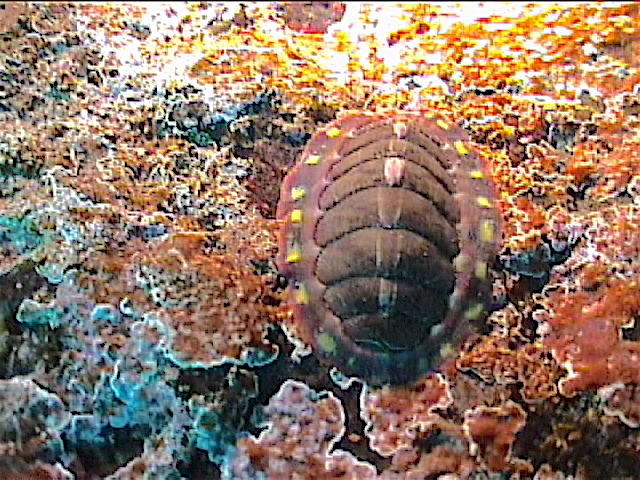The image shows a blurry and distorted photograph, likely a screenshot from a video, depicting an underwater scene with intricate details. At the center, there is an object that resembles the back of a turtle, characterized by a dark brown shell with slight humps lining its center. This shell is adorned with a pattern of yellow rectangles or polka dots along the edges. The surrounding environment is a complex array of red, orange, and rust-colored coral or reef-like formations, which densely populate the scene, making the water itself barely visible. These formations are detailed with white streaks, and various sections of the image also showcase light blue, gray, and black hues, particularly towards the corners. The overall scene has an infrared-like quality with vivid reds and purples popping against the darker background.